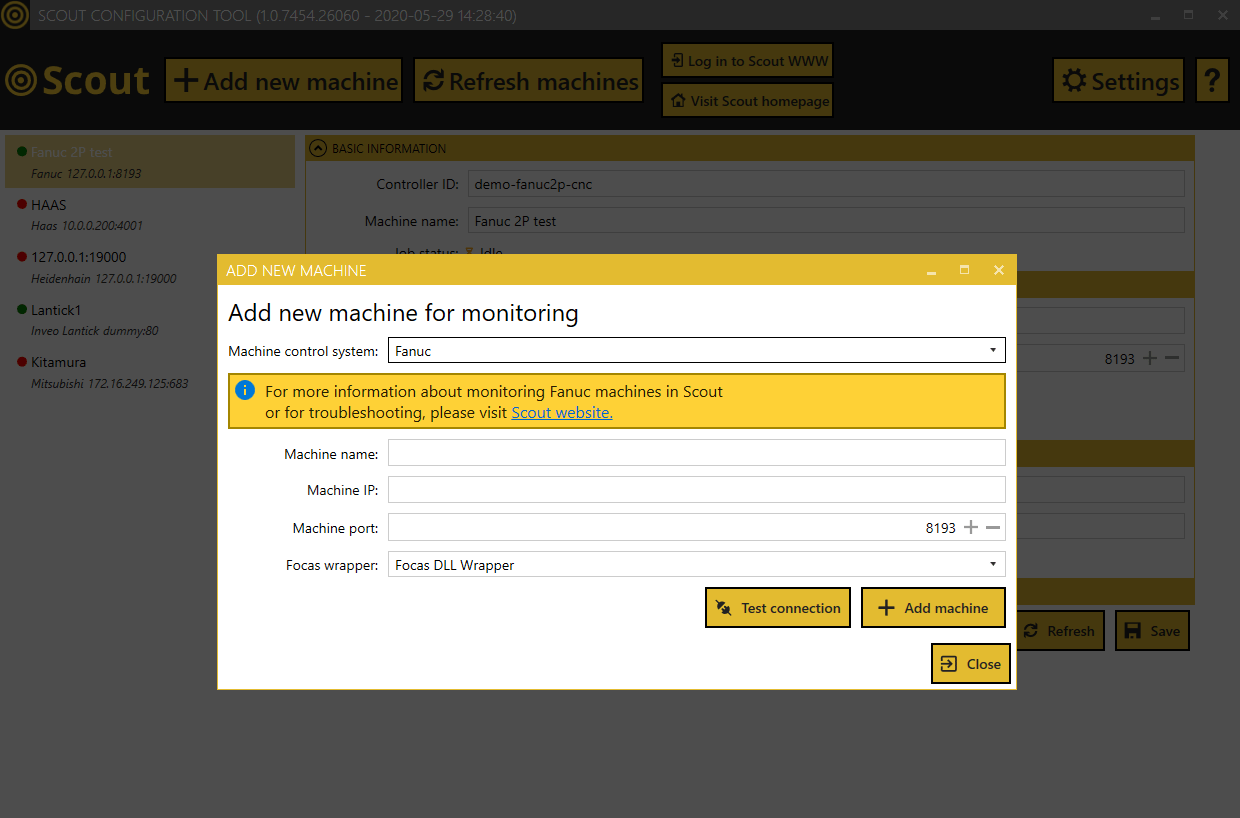**Descriptive Caption:**

The image displays a main web page that is grayed out and de-emphasized because a prominent pop-up window is in focus at the center of the screen. The background of the main web page is primarily white, with a noticeable yellow banner at the top. This banner contains the bold text "Add New Machine."

Below the banner, the pop-up window is divided into various sections. At the top of the pop-up, it reads "Add New Machine for Monitoring," accompanied by a form field labeled "Machine Control System." A drop-down box next to this field has "F-A-N-U-C" selected.

Directly beneath the form field, a horizontal yellow information banner spans across the pop-up. In the upper left corner of this banner, there is a small blue icon with a white "I" in its center, indicating an information sign. The accompanying text on the banner provides guidance: "For more information about monitoring F-A-N-U-C machines in Scout, or for troubleshooting, please visit the Scout website."

Below the information banner, the form continues with several fields designed to input details about the new machine. These fields are labeled as "Machine Name," "Machine IP," "Machine Port," and "Focus Wrapper." The "Focus Wrapper" field is a drop-down menu with "Focus DLL Wrapper" selected.

At the bottom right of the pop-up window, three yellow buttons are lined up horizontally. They are labeled "Test Connection," "Add Machine," and "Close," providing different actions for the user to perform regarding the new machine setup.

Overall, the pop-up window is central, fully detailed, and contains a combination of explanatory text, form fields, and actionable buttons to assist in adding a new machine to the monitoring system.